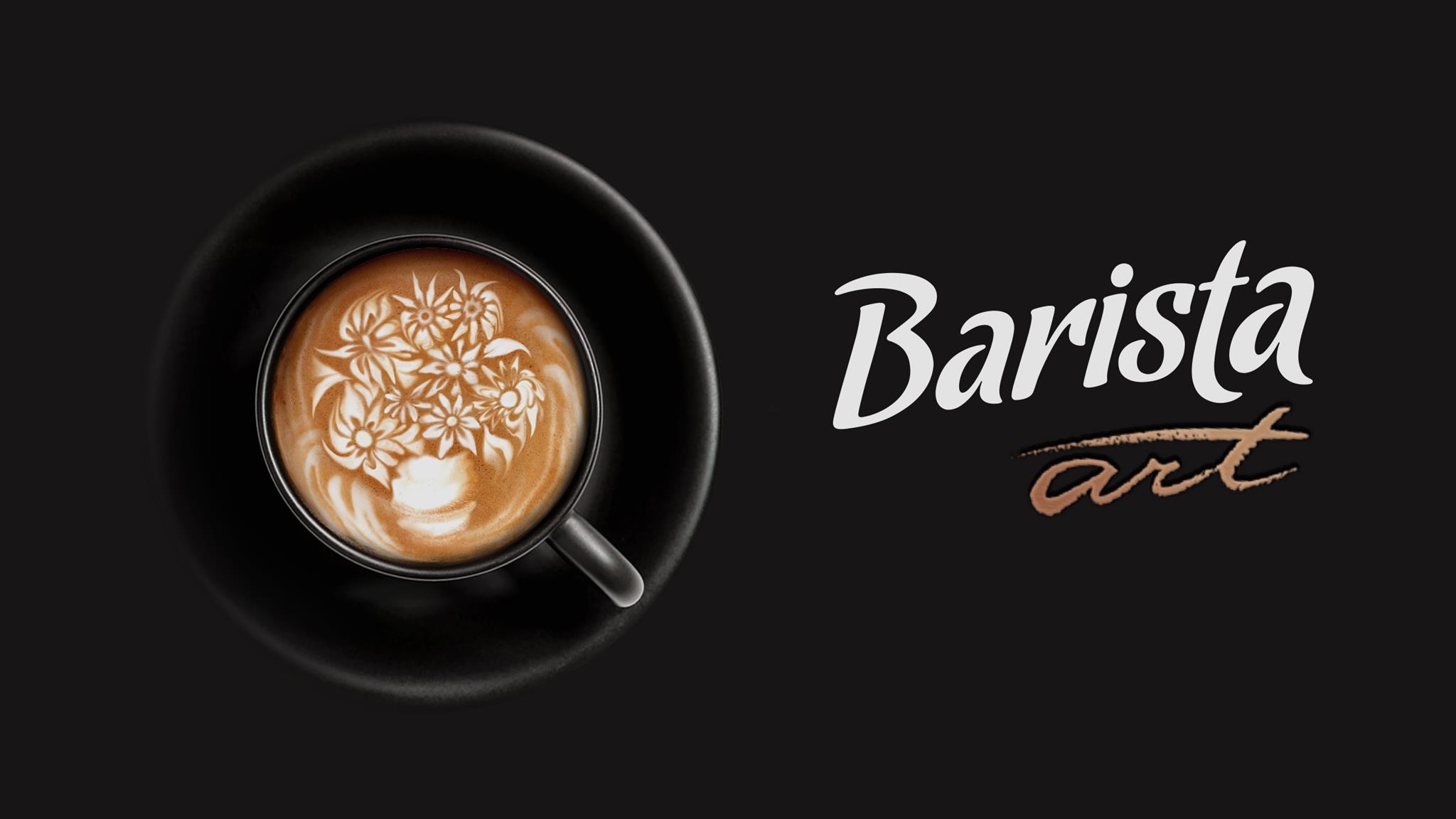The image is an advertisement featuring a black background. At the center-left of the image, there is a top-down view of a black cup of coffee resting on a matching black saucer. The cup showcases an intricate barista design on the coffee's surface, which artfully depicts a vase holding multiple flowers in full bloom, complete with detailed petals and accent lines. To the right of the cup, in diagonal alignment, the word "barista" is prominently displayed in white text, followed by the word "art" in brownish cursive text, slightly rising upward from the left to the right. This impressive artistic creation, presumably made with cream, highlights the skill and pride of the barista who crafted it.